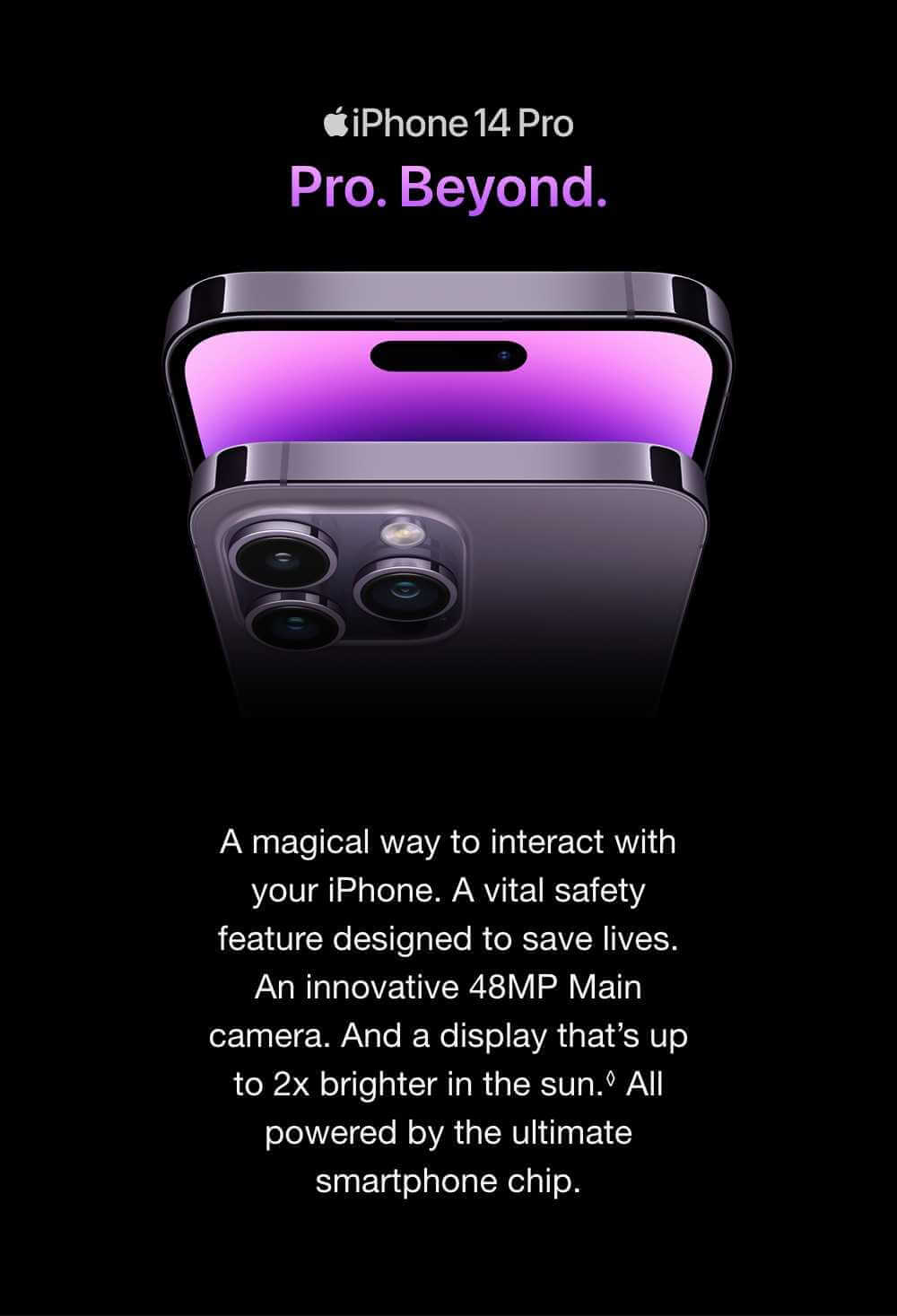This is a detailed screenshot of an advertisement for the iPhone 14 Pro. The background is predominantly black, with the Apple logo displayed at the top in gray. Below the logo, the phrase "Pro. Beyond." is prominently featured in purple letters. Beneath this bold statement is an image showcasing both the front and back of the iPhone 14 Pro. 

The back of the phone highlights its triple-camera system accompanied by a flashlight. The front display is vibrant in purple, with sleek, shiny edges giving it a luxurious appearance. Further down the page, a descriptive text in white reads: "A magical way to interact with your iPhone. A vital safety feature designed to save lives. An innovative 48-megapixel main camera and display that's up to two times brighter in the sun. All powered by the ultimate smartphone chip."

This concise yet comprehensive advertisement page expertly captures the innovative features and premium design of the iPhone 14 Pro.